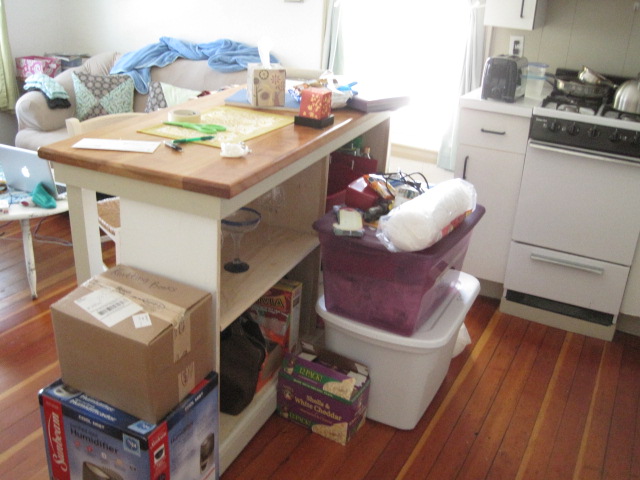This detailed photograph captures a bustling kitchen space with a prominent central island. The kitchen island, equipped with shelves, is cluttered with various items including pens, papers, and boxes. One shelf hosts an array of glassware, while the shelf below stores food items like cereal and noodles. Surrounding the island are numerous boxes and totes, filled with miscellaneous objects, adding to the sense of activity and storage.

Beyond the island, the expected dining area features an unusual setup with a sofa and a short coffee table, atop which rests an open Apple laptop, suggesting a casual, multipurpose use of the space. In the kitchen area itself, a narrow gas stove is prominently placed, heavily laden with pots and pans, highlighting ongoing culinary activity. Adjacent to the stove is a toaster. The cabinetry encasing the kitchen is white, contrasting with the white and black-trimmed range, contributing to an overall sense of a lived-in and dynamic household.